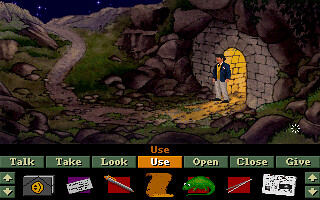The image is a screenshot from an adventure story video game, featuring an intricate menu of gameplay options. From left to right, the menu options displayed at the bottom of the screen are: Talk, Take, Look, Use (highlighted in white font on a gold background), Open, Close, and Give. Below the menu, there are various rectangular icons, including a pen, a scroll, a book with a yellow smiley face, a purple, white, and black object, a red sheet of paper, a green animal, a red square, and some white papers.

The central image showcases a well-dressed man, clad in a dark coat, yellow shirt, light pants, and black shoes. He stands outside a stone doorway, reminiscent of a cave entrance, with a golden light emanating from within. The scene is set against a backdrop of a dirt path bordered by grass and scattered stones, with a hint of the night sky above. The attention to detail in both the character’s attire and the surrounding environment gives the image depth and immersiveness, characteristic of the genre.